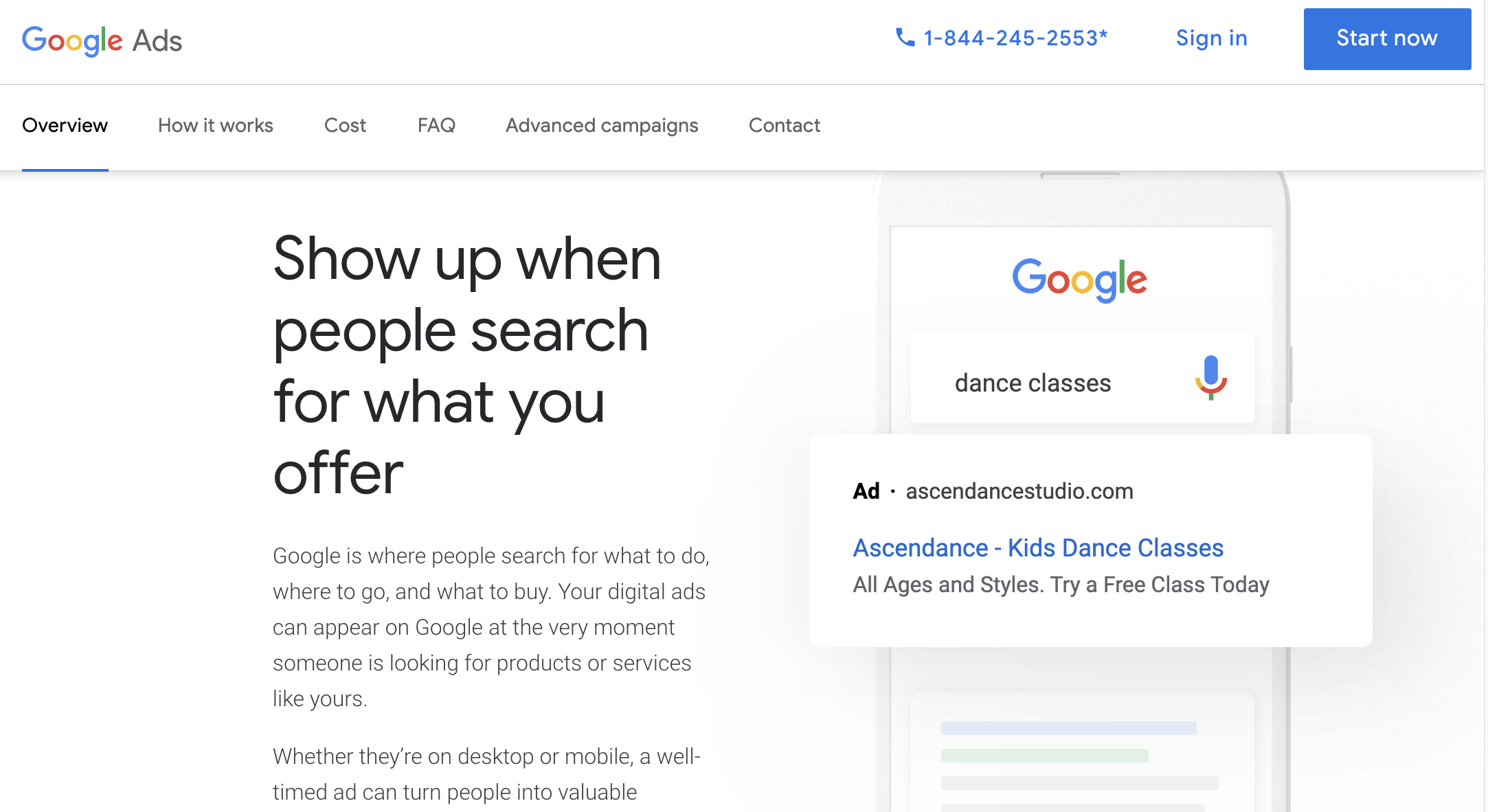This screenshot appears to be from a computer displaying a Google Ads page. At the top left, the text "Google Ads" is prominently featured, accompanied by a customer support number, 1-844-245-2553. The page offers options to "Sign In" or "Start Now," indicating entry points for users.

The central message of the page reads: "Google Ads: Show up when people search for what you offer," suggesting it is a platform where businesses can purchase advertising space on Google. Beneath this overview, there are tabs titled: Overview, How it Works, Cost, Frequently Asked Questions, Advanced Campaign, and Contact. These tabs likely provide detailed information and guides for setting up and managing Google Ads.

The detailed description emphasizes that Google Ads can make businesses' digital advertisements appear precisely when users search for related products or services. This functionality can effectively convert searches on desktop and mobile devices into valuable engagements for advertisers.

To the right of the main text, there's an example ad showcasing a business named "AscendanceStudio.com," which promotes "Ascendance Kids Dance Classes: All ages and styles, try a free class today." This ad serves as a visual example, demonstrating what a live Google Ad might look like, potentially reflecting an ad created by the dance studio owner currently on the page.

Overall, this screenshot represents a Google Ads informational and setup page designed to attract and guide potential advertisers in creating effective digital ad campaigns.